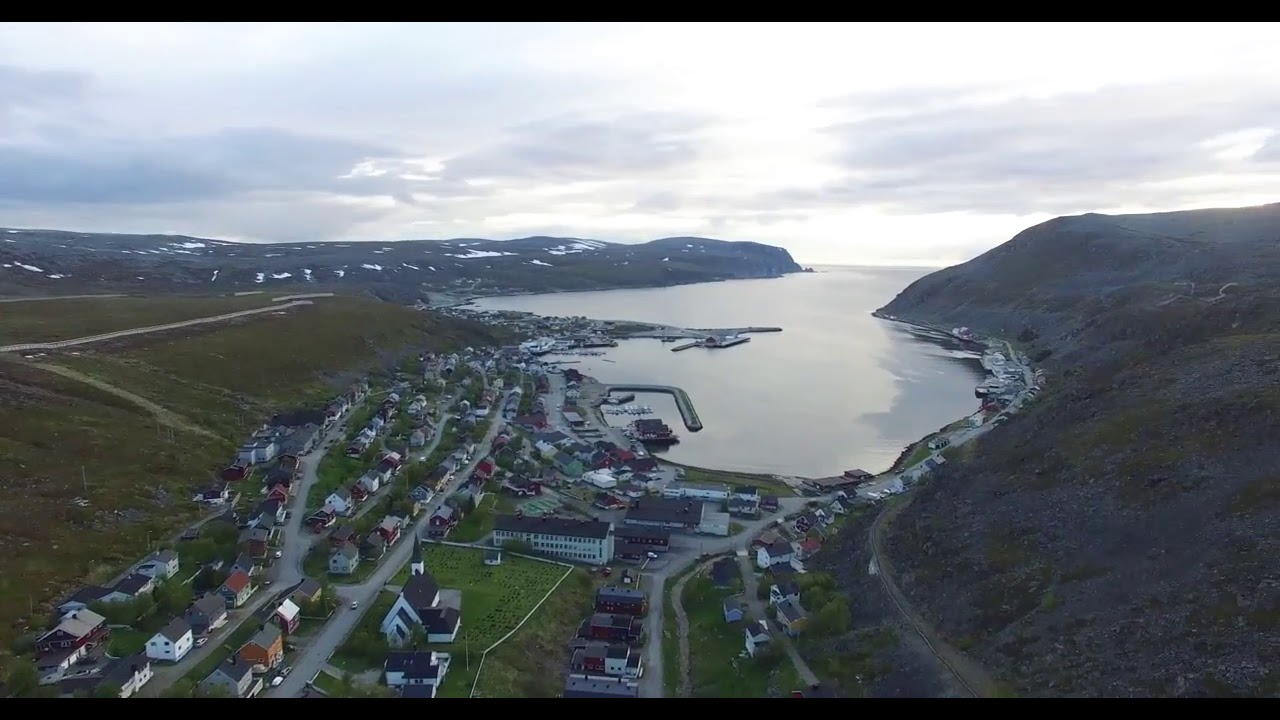The photorealistic image presents an aerial view of a serene small town nestled by a bay. Rich green grass blankets the area, contrasting with the concentrated cluster of dozens of small buildings near the bottom center of the image. These buildings, characterized by dark-colored roofs and bright walls in hues like white, red, and gray, are crisscrossed by numerous gray roads. The focal point of the town extends down to a small bay, centrally positioned, with its gray water gradually opening into a larger body of water toward the right side.

The bay is adorned with several docks, extending outward, some hosting parked boats. To the right and left of the image, as well as in the background, imposing hills rise majestically. They display a mix of dark gray, green, and brown hues and are speckled with patches of snow. These natural elevations envelop the water, creating a somewhat enclosed feel.

In the distance, the sky transitions into a gradient of gray-blue, dominated by dark clouds that add a somber tone to the scene. The town's layout extends from the left towards the bottom center, showcasing a mix of tightly packed rows of homes and open green spaces, possibly yards or play areas. The overall image encapsulates a tranquil maritime village, surrounded by encircling hills and crowned by a broody sky.